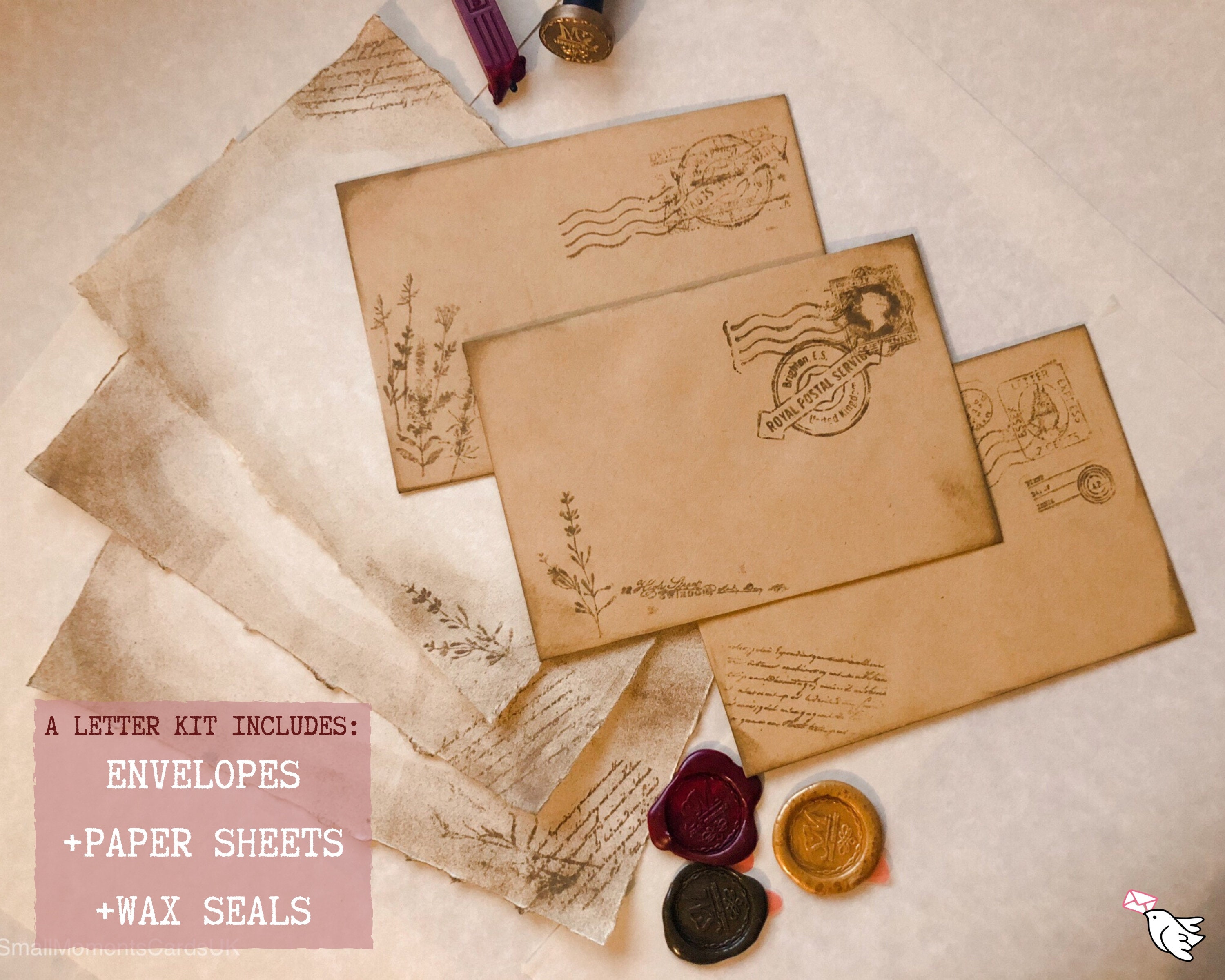This detailed image showcases a vintage-style letter kit meticulously arranged on a pale brown, parchment-like surface. At the center, three antique brown envelopes, each stamped in the upper right-hand corner, are staggered on top of one another. To the left, three sheets of parchment paper, also brown and worn with smudged corners, lie beneath each other, featuring delicate leaf and stem stamps. Prominently positioned at the top, a small circular gold wax seal stands out, with a stick of purple wax nearby. At the bottom, three wax seals in purplish-red, gold, and green are displayed, showing intricate stamping work. In the lower left corner, a light pink square contains a label in dark pink lettering that reads "A Letter Kit Includes," followed by white text listing "Envelopes, plus Paper Sheets, plus Wax Seals." The lower right corner features a white bird clutching an envelope, tying together the cohesive and nostalgic theme of the Royal Postal Service-inspired kit.